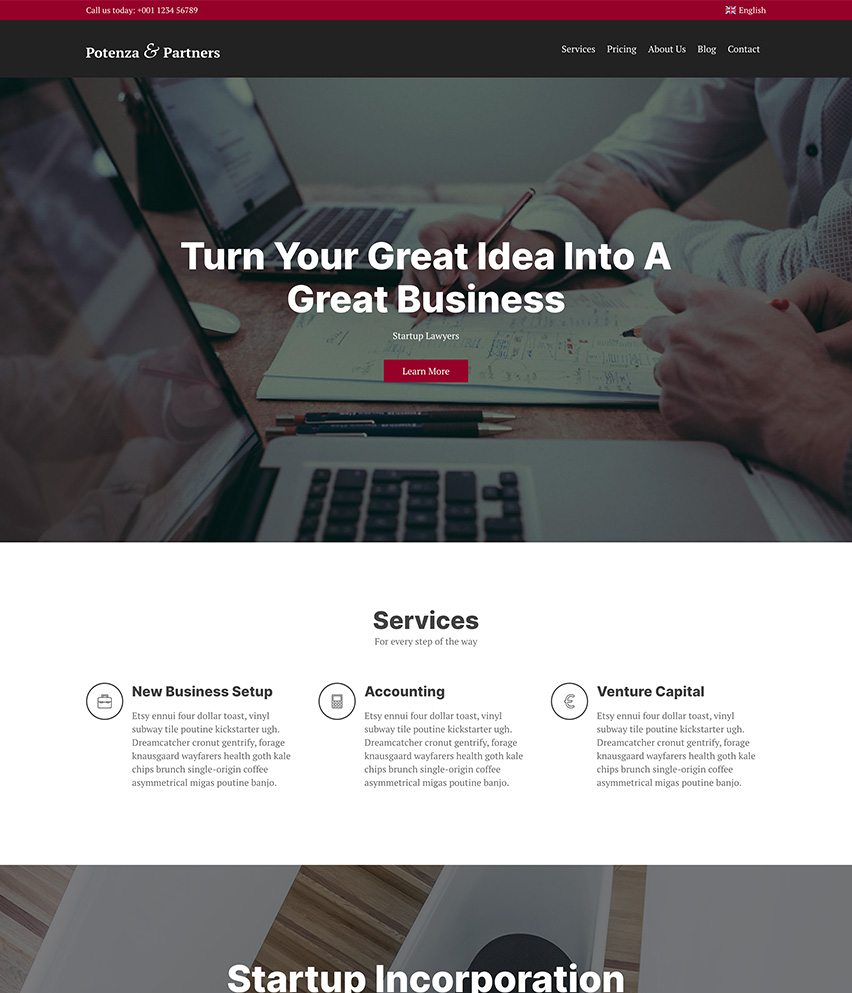In this detailed image, viewers are presented with the homepage of the Potenza and Partners website. The top right corner features a button for changing languages, currently set to English. The website's navigation bar on the right side displays icons or buttons for various sections: Services, Pricing, About Us, Blog, and Contacts. The central text on the homepage encourages visitors to "Transform your great idea into a great business," highlighting the firm's focus on start-up support with a call to action button labeled "Learn More."

The page further outlines the array of services offered, under the slogan "Services for every step of the way," which include New Business Setup, Accounting, Venture Capital, and Startup Corporation assistance. The color scheme of the page prominently features shades of white, red, and black, enhancing the professional and dynamic aesthetic of the website.